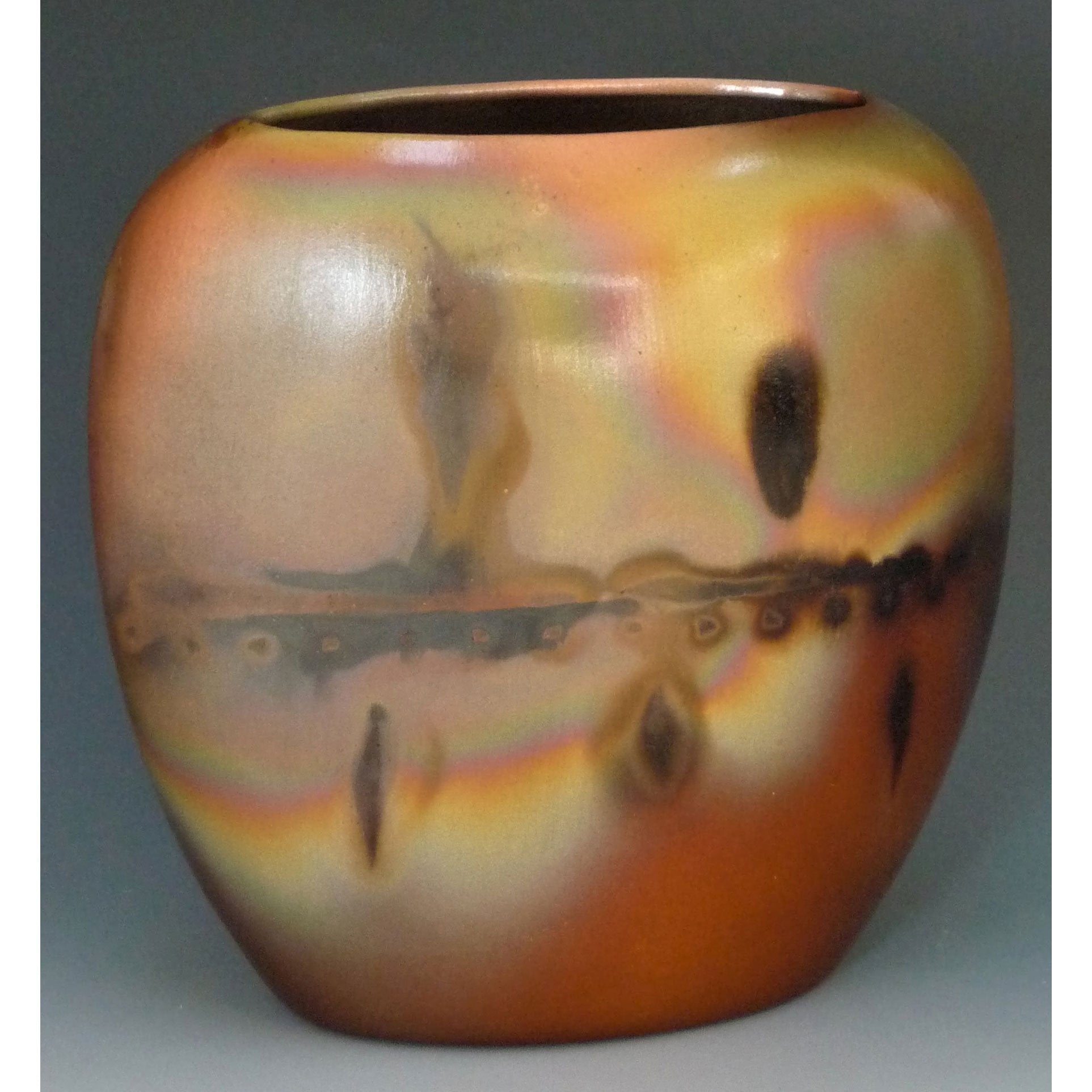The photograph captures a large, historically-styled ceramic vase displayed against a dark gray background that lightens towards the bottom. The vase, which could be the size of a watermelon, has an imperfect, ovular shape, reminiscent of an apple with the top cut off. Its base color is a dark orange or brown, transitioning into a washed-out, rainbow-tinted pattern towards the top. These rainbow hues include yellows, greens, blues, and purples, resembling the effect of splashed water on wet paint. The vase has a central line dividing it, with small circles below this line and larger circles both above and below it. The surface of the vase has a burnt appearance with scorched marks, making it look somewhat like fuel spillage on asphalt under sunlight. The central opening of the vase is circular and black. This professionally photographed piece, possibly a museum collection item, exudes a sense of historical and aesthetic significance, despite—or perhaps because of—its imperfections.